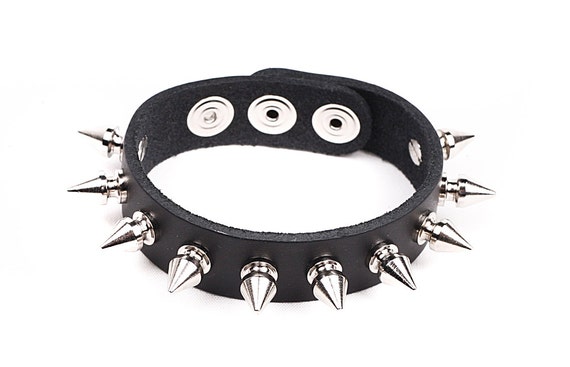A detailed photograph showcasing a spiky, metal, gothic-style black bracelet. The black strap, adorned with approximately ten half-inch metal spikes, rests on a stark white surface. The image is taken from an overhead perspective, revealing both the exterior and interior of the strap. The blunt, cylindrical spikes are securely affixed to the strap, reinforcing the rugged aesthetic. The backside of the bracelet features three metal snap buttons for adjustable wrist sizing, currently fastened at the middle button to accommodate a medium-sized wrist. The minimalist background ensures that the striking design and craftsmanship of the bracelet remain the focal point of the image.